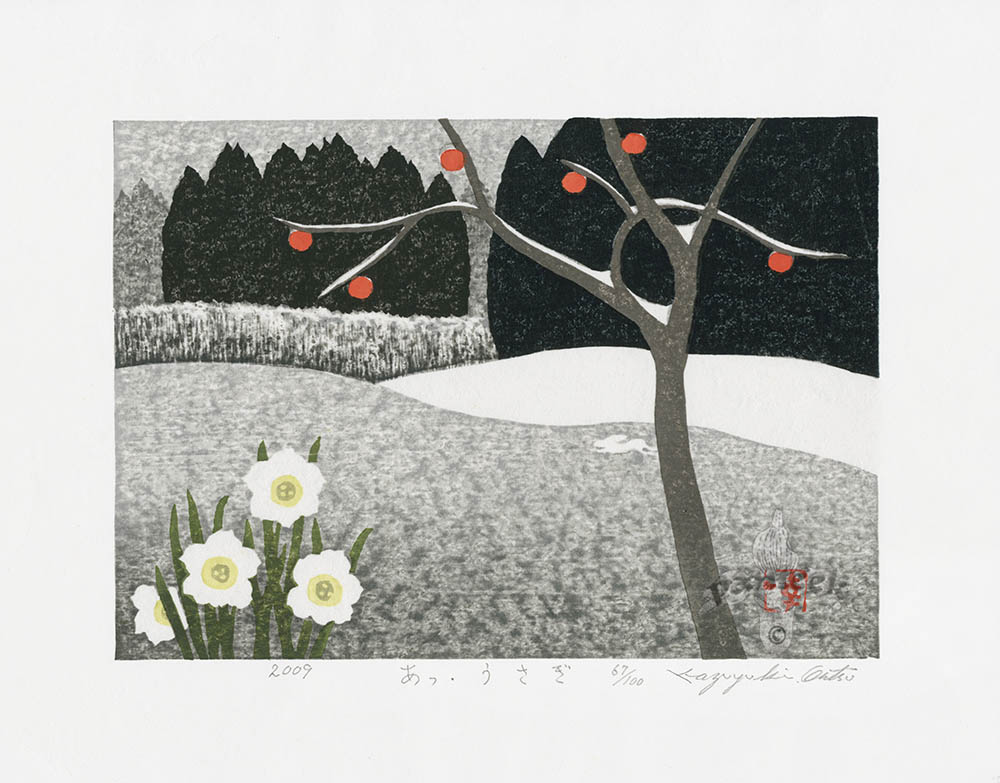This is a detailed painting, likely a digital print, illustrating a somewhat abstract winter landscape. The scene is primarily rendered in grays, whites, and blacks, with a few vibrant bursts of color. The foreground features a bare tree with six bright red fruits, possibly berries or small oranges, clinging to its branches, which also have patches of snow nestled in their crotches. Nestled in the bottom left corner is a cluster of white daffodils with yellow centers and green leaves, providing a lively contrast to the muted tones. The background reveals the outlines of dense, dark pine trees silhouetted against a gray sky. Rolling hills stretch across the scene, one gray in the front and a snowy white one to the right. A notable feature is a small, white rabbit in motion, located near the tree. Additional details include "2009" inscribed in gray text at the bottom, the artist's partially legible signature starting with a "P", and a watermark that says "Pantique" accompanied by a red Japanese stamp. The entire image is bordered by a large white matting, giving it a clean, framed appearance.